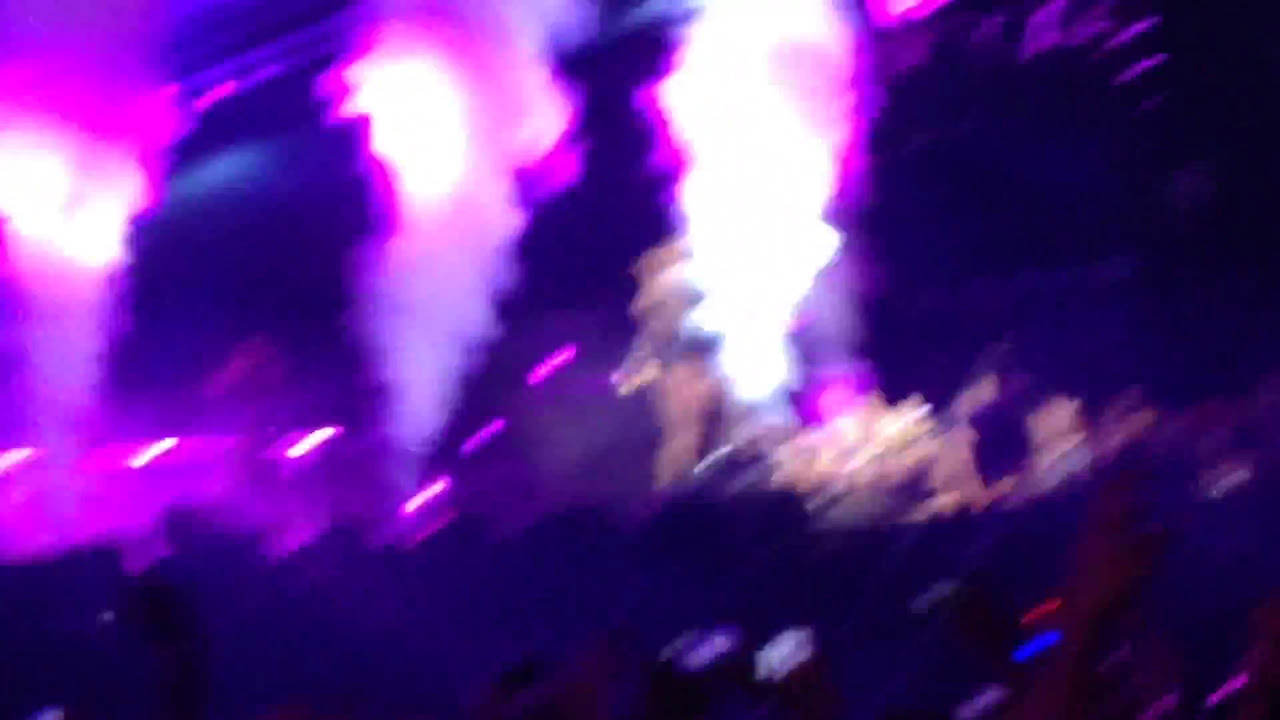This is a blurred photograph taken inside a dark venue, likely a concert. The main colors are a mix of blue, purple, pink, and black, with areas of white and red. In the foreground, there appear to be hands raised in the air, suggesting an enthusiastic audience facing a stage. The image is very hazy, with a potential performer vaguely visible amidst the blur. Distinctly, there are three areas from which flames or smoke seem to be emanating, characterized by a blend of white, red, grey, lavender, and magenta tones. Midway up the picture, there are blurry fluorescent lights casting a pink and purple glow. The overall scene is dynamic and chaotic, capturing the energetic atmosphere of a live performance.